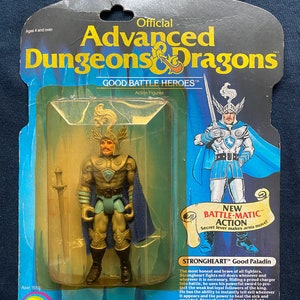This is an image of a low-resolution, packaged action figure being sold, likely on platforms such as eBay or Etsy. The figure is an official Advanced Dungeons & Dragons collectible labeled "Goods Battle Heroes." The packaging, designed for hanging on a store peg, prominently features "Official Advanced Dungeons & Dragons" in bold, yellow print over a blue background, with the name "Good Battle Heroes" noted above. The plastic encased figure, identified as "Strongheart TM," depicts a male paladin adorned in detailed gear: a winged helmet with a high plume, a blue cape, silver armor, tight silver leggings akin to He-Man, and cropped blue armor. Additionally, he wields a sword included in the package. The packaging also showcases a cartoon drawing of the figure on the side, highlighting "New Battlematic Action." The backdrop of the plastic casing includes green and yellow tones, setting off the character's detailed armor and accessories against a black package background.